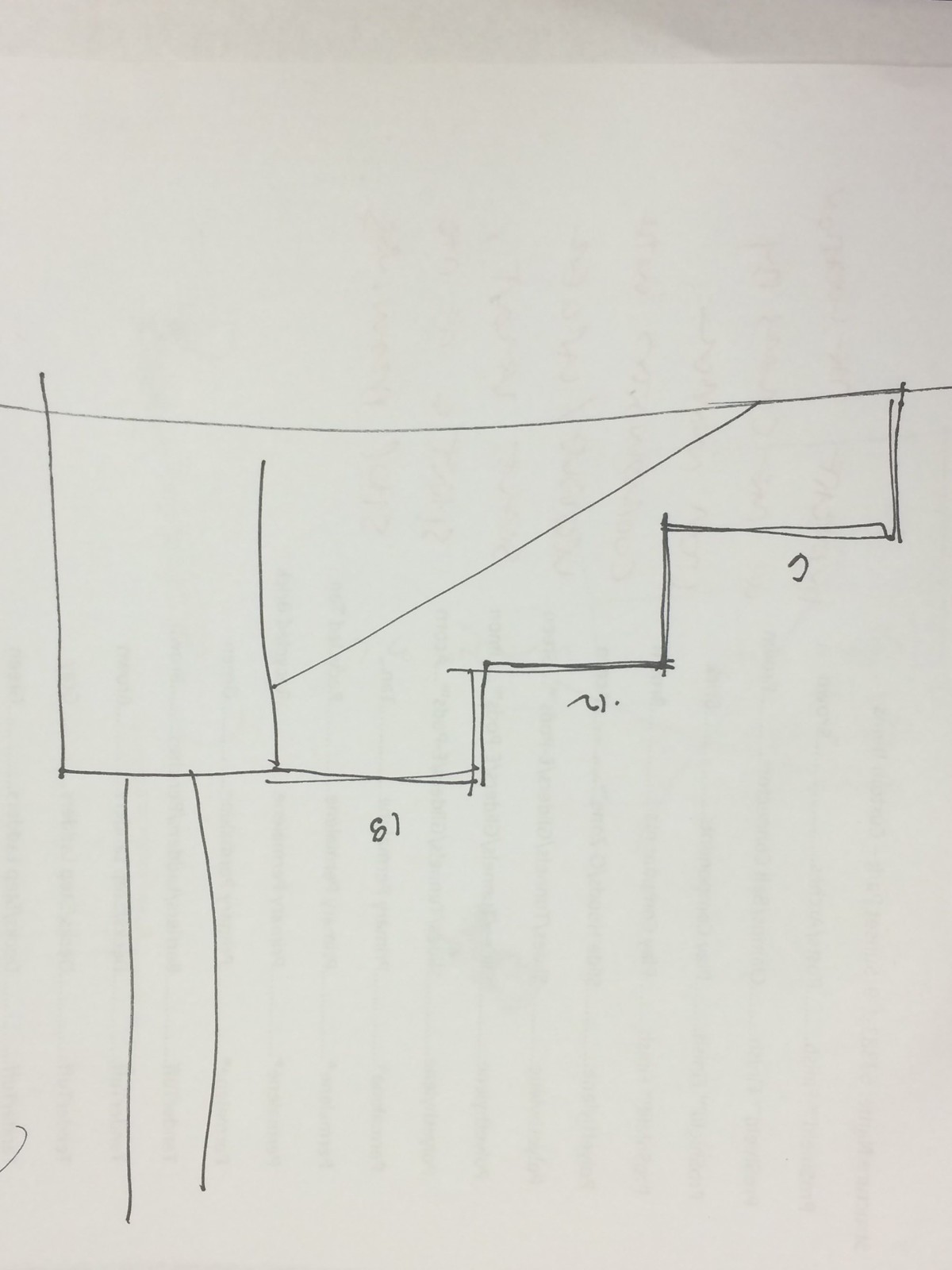This drawing appears on a piece of white, possibly professional drawing paper or regular typing paper that has been repurposed. The paper shows signs of previous use, with visible vertical streaks indicating it had been folded or marked earlier. The drawing itself, executed entirely in pencil, depicts what seems to be shelving units or a series of steps arranged upside down. 

The composition features a straight edge at the top and left sides, while the right side includes a series of lines forming a stepped pattern: approximately two inches down, three inches across, then another two inches down and an inch sideways, before extending all the way across. Below these steps, there are some numbers inscribed—possibly indicating measurements or labels—showing "6" on the first step, "12" on the middle step, and "18" on the last step. There is some ambiguity as these might also read "81," "21," and "0," depending on the orientation of the drawing.

Additionally, a diagonal line spans from the first step to a point approximately a quarter of the way from the left edge of the paper. Beneath the left-hand edge, two vertical lines extend downward, perhaps suggesting an entryway. The drawing could be an architectural sketch, possibly outlining the design for stairs, cabinets, or another structural element.